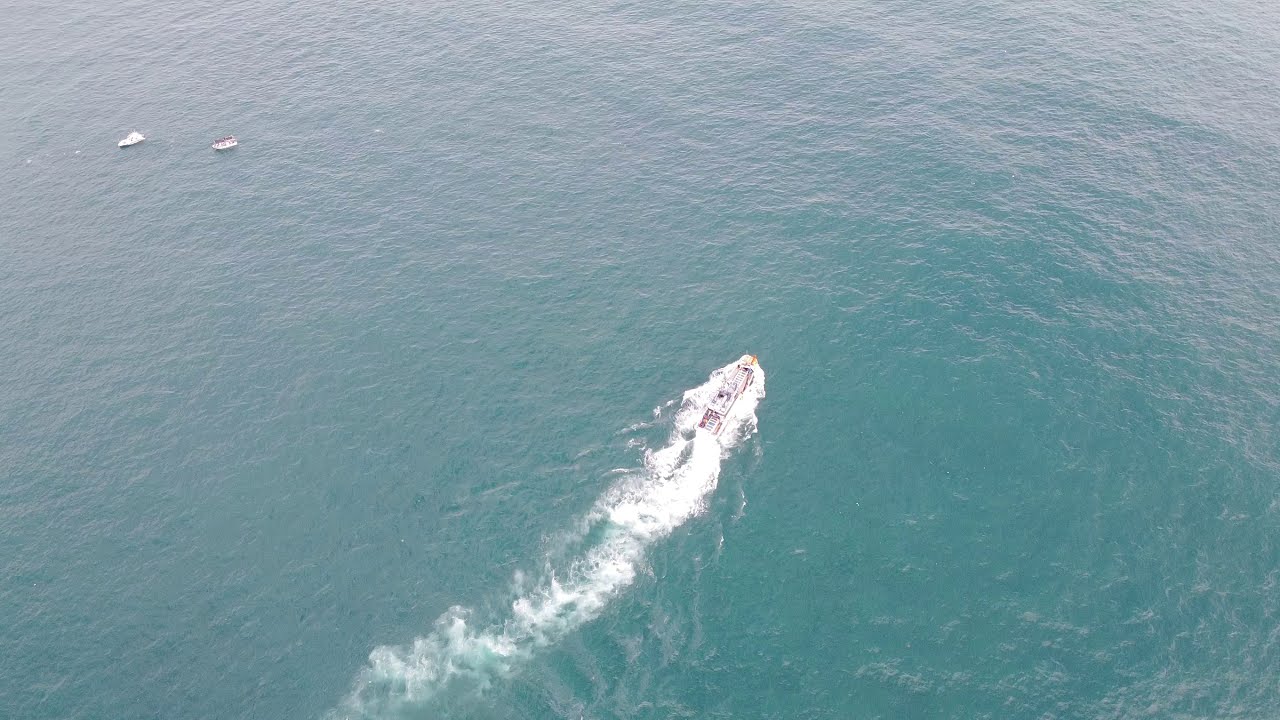This is a color landscape-oriented, aerial photograph depicting a vibrant ocean scene. The image, taken from well above, showcases a large white speedboat prominently centered and moving diagonally from left to right across the frame, leaving a distinct wake of white foam in its path. The water, a striking aqua blue, spans the entire background of the photograph, creating a serene and expansive setting devoid of any visible land or sky. In the top left-hand corner, two much smaller white boats can be seen, adding a sense of scale and motion to the composition. The detailed realism of the photograph offers a clear and vivid representation of this maritime scene.